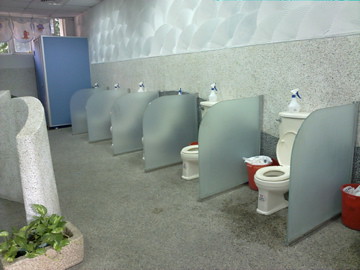This image depicts a uniquely designed public bathroom with several distinctive features. The room has a grey speckled stone wall that transitions midway to textured drywall. Arranged in a diagonal line from the right to the left corner are five white toilets, each separated by semi-translucent glass partitions without doors or tops. The toilets feature red trash cans positioned beside them, and on the back of each toilet tank are white squirt bottles with blue handles. 

In the far left corner is a tall, blue shelving unit. At the bottom left corner of the image, a rectangular stone planter filled with green-leafed vines can be seen. Behind this planter, a curved faux stone partition wall extends to the left, out of the frame. The ceiling of the bathroom is painted blue, complementing the blue shelving unit at the back. The setup creates a visually cohesive and distinctively organized bathroom space.